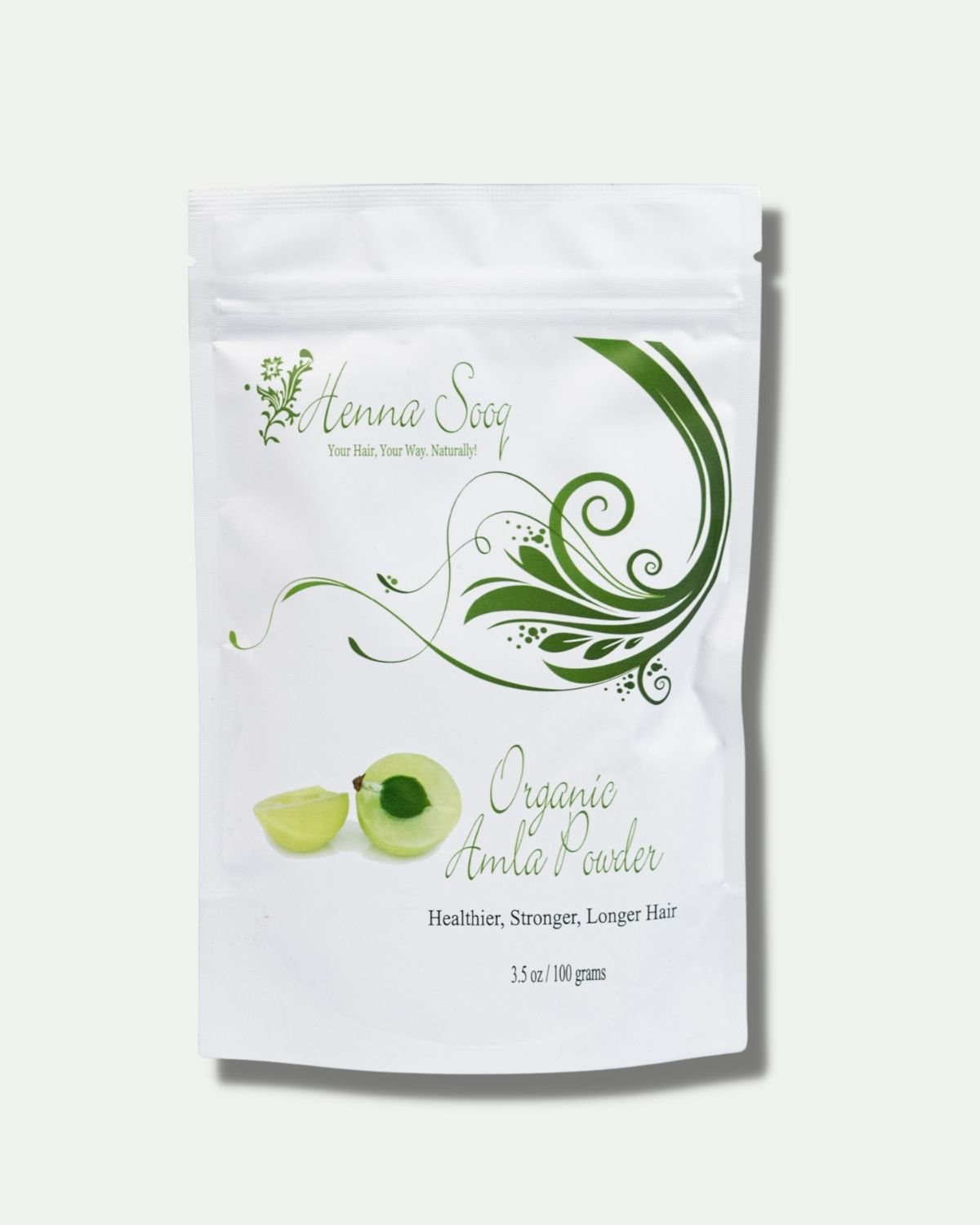The image is a professionally taken overhead photograph of a white, resealable pouch of Henna Sooq Amla Powder, designed to promote healthier, stronger, and longer hair. The front of the package, which is taller than it is wide, features green lettering and decorative elements, including an artistic leafy design to the left of the product name and an intricate filigree to the right. Prominently displayed near the top is the brand name "Henna Sooq," followed by the slogan "Your hair, your way, naturally." Below this, it states "Organic Amla Powder" and vividly depicts an open avocado with a dark green pit. The package, containing 3.5 ounces (100 grams) of powder, is placed on a white background that has a very subtle light green tint. This minimalist setup emphasizes the product, making it the clear focal point of the image.